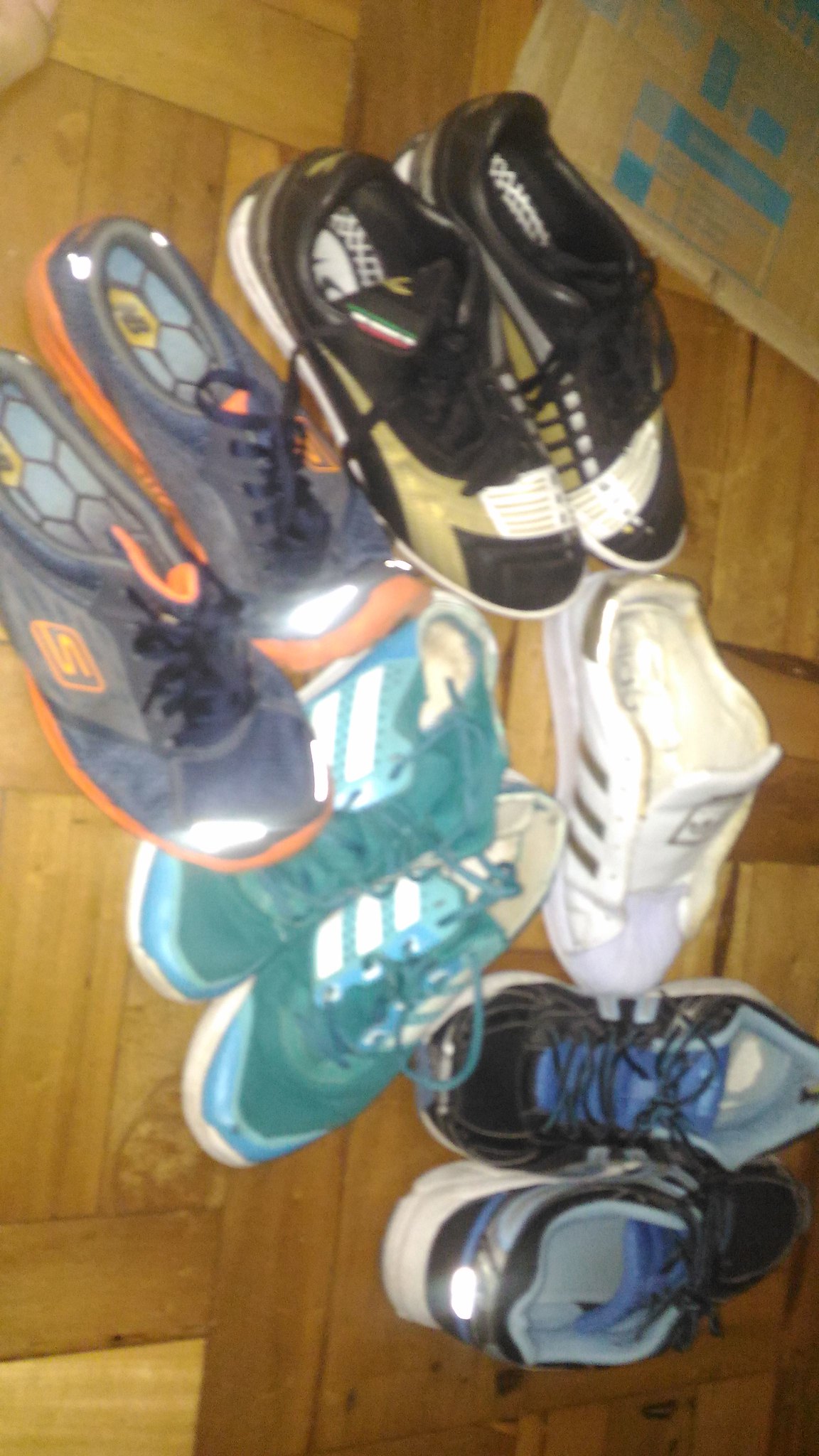This image features an assortment of sneakers arranged haphazardly on a light-colored wooden parquet floor. In the upper left corner, a cardboard box with blue markings is partially visible. The sneakers include four complete pairs and a single mismatched shoe without its mate. The top pair is black with white and tan accents, while the pair to the left is gray and orange with dark laces, featuring an orange S logo and reflective spots at the toes. Below those, there is an aqua and teal pair with white soles and three stripes on the side. Directly beneath these, there is a pair of black and blue sneakers with two stripes and a reflective spot on the back. The lone shoe among the collection is white with black stripes, its tongue prominently pulled up and lacking visible laces. The shoes are arranged facing various directions, adding to the sense of casual disorder.